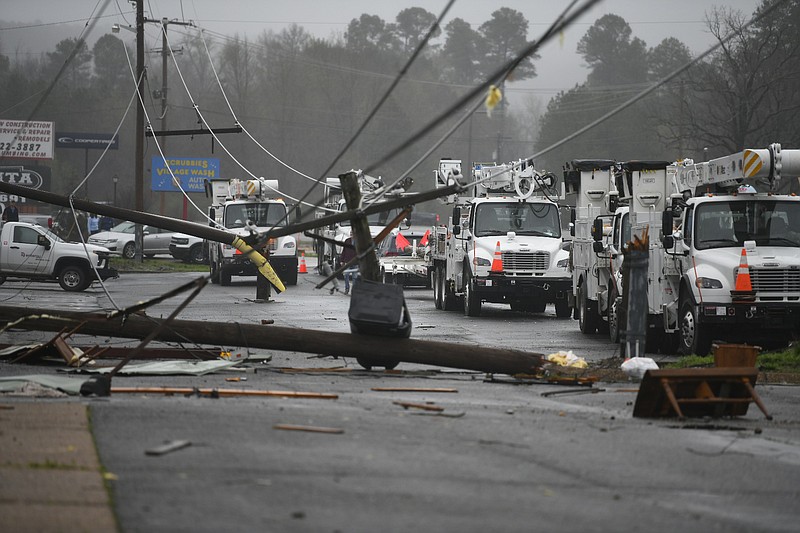The image depicts a chaotic scene of what appears to be storm or accident damage, set against a gray, overcast sky. In the foreground, a toppled electrical pole lies across a wet, gray street, with a tangle of wires strewn in various directions. Multiple utility trucks are lined up, equipped with bucket ladders and orange cones, ready to address the damage. A total of at least four trucks, possibly more, extend from the middle right to the middle left of the image, reflecting their readiness to tackle the mess. Background elements include various business signs, trees, and additional wreckage, suggesting extensive disruption. Among the debris, there appears to be a fallen traffic light or pedestrian signal and other scattered objects. The overall impression is one of significant roadway disruption, likely caused by a severe storm or major accident, with utility crews actively engaged in restoration efforts.